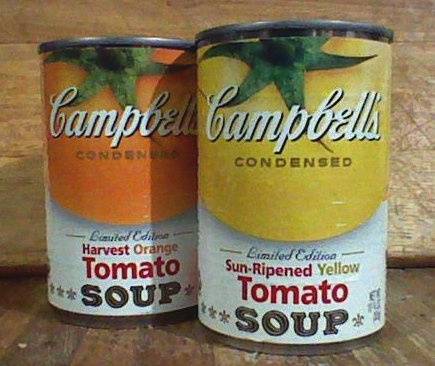This image showcases two vintage-style Campbell’s soup cans positioned at the center. The photograph is in color and taken in landscape format. Both cans exhibit a nostalgic design characterized by a classical font and unique coloring, enhanced by a distinctive border around the top not seen in modern products. The cans sit on a dark brown wooden surface against a lighter brown wooden wall backdrop.

On the left, the can features an orange tomato with a green stem and is labeled "Harvest Orange Tomato Soup" in red and orange text. Next to it, the right can displays a yellow tomato with a green stem, identified as "Sun-Ripened Yellow Tomato Soup" in red and yellow text. Both cans bear the "Campbell's" brand name prominently in white with black outlines at the top, followed by the word "condensed" underneath, and the word "soup" in gold and black at the bottom. These cans are special limited editions, adding to their unique vintage appeal.